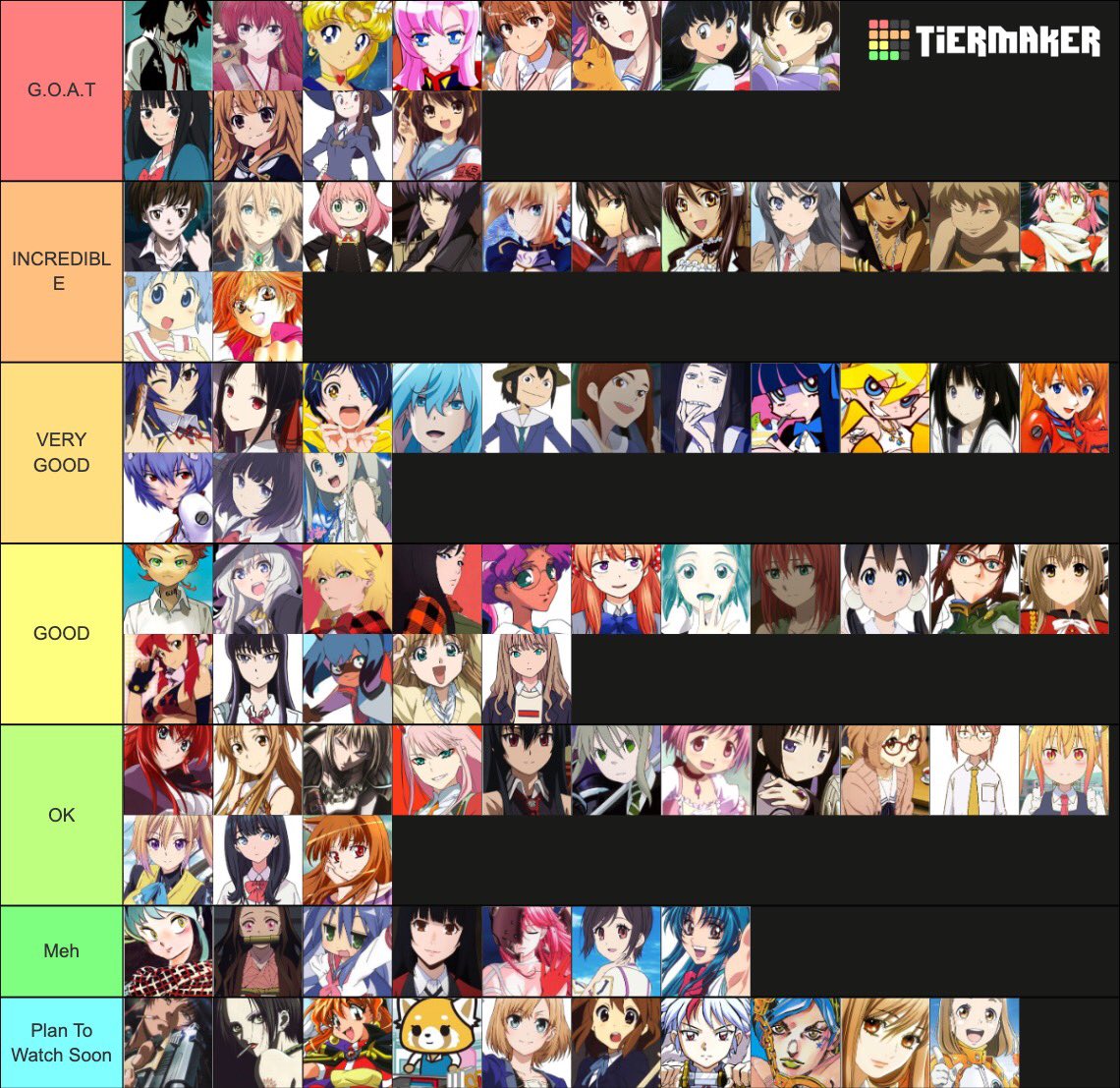The image is a tiered ranking of anime characters, created using TierMaker, a program that lets users rank various items. At the top right corner of the image, "TierMaker" is displayed in white blocky letters next to a logo featuring two red squares, four orange squares, two yellow squares, and three green squares. The rankings are color-coded and divided into several categories:

1. **G.O.A.T. (Greatest of All Time, in red)**: This top tier contains the most esteemed characters and features eight images of primarily female anime characters.
2. **Incredible (muted orange)**: This tier showcases a highly-rated selection of anime characters.
3. **Very Good (dark yellow)**: A tier for characters considered very good includes numerous images.
4. **Good (yellow)**: Contains multiple pictures of anime characters rated as good.
5. **Okay (light green)**: This tier ranks anime characters that are okay, with several images.
6. **Meh (medium green)**: A smaller category for characters deemed meh.
7. **Plan to Watch Soon (light blue)**: At the bottom, this tier includes anime characters the creator plans to watch soon, featuring a mix of colorful designs including a raccoon.

Overall, the tier list visually organizes a diverse array of anime character faces in a detailed and colorful manner.